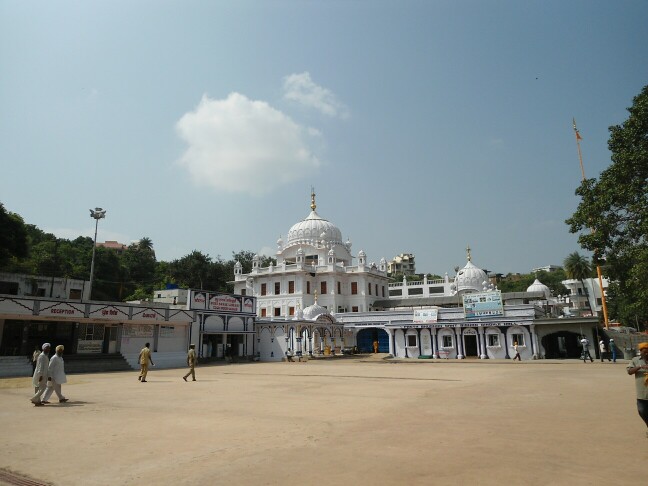The photograph depicts an outdoor scene on a rectangular property that is reminiscent of a religious site, likely in India, characterized by its vast open courtyard. Encircling the beige, smooth courtyard is an ornate white building embellished with gold accents, suggestive of a temple or significant cultural structure. The building features rectangular windows, small columns lining the roof, and a large central dome with a gold steeple, rising to about three stories high. Flanking the main structure, there are extensions that give the appearance of offices, one of which is marked with a sign indicating "reception." The sky above is a clear blue, punctuated by a couple of fluffy white clouds, and significant tree lines border the property in the background. Within this serene setting, several people dressed in traditional Indian garb, including turbans and other attire often associated with Sikh men, can be seen walking around the courtyard, adding a vibrant cultural touch to the scene.